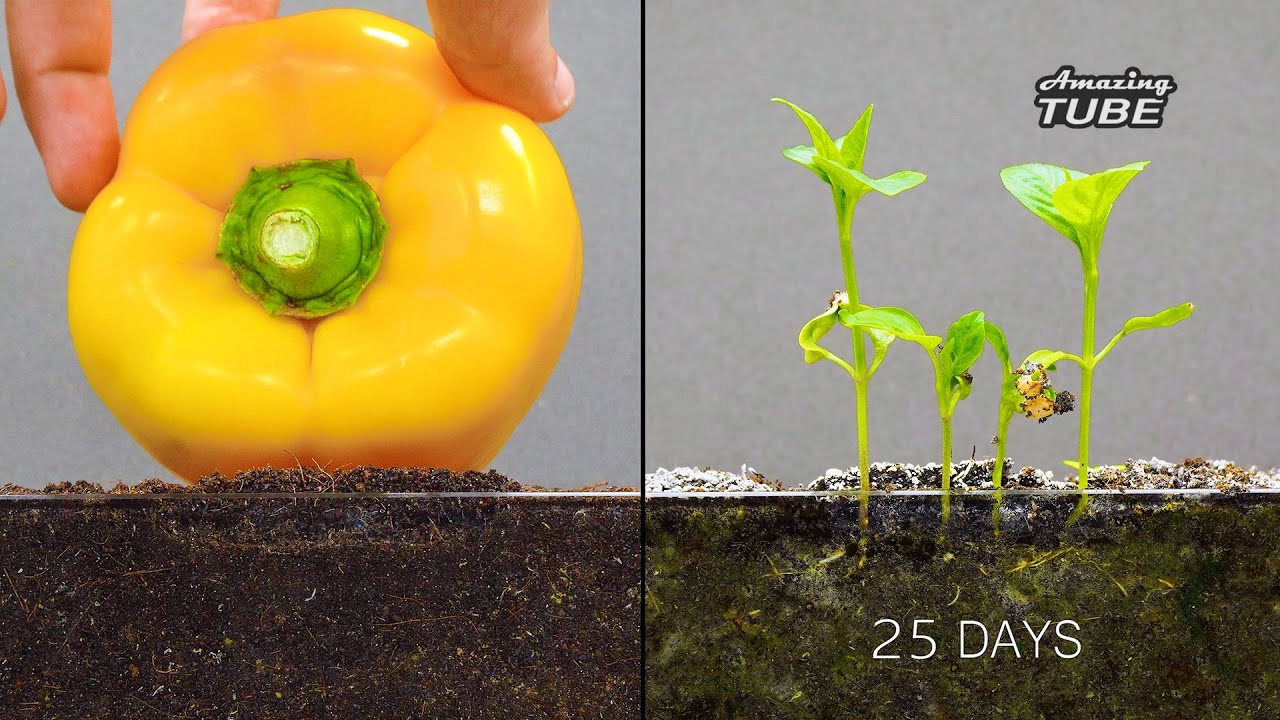This image presents a two-part scientific diagram illustrating the growth stages of a yellow bell pepper plant. On the left, a close-up shows the fingertips of a person holding a yellow bell pepper horizontally, with the stem facing forward, partially submerged in a layer of soil. On the right, the second image captures the same soil 25 days later, where four green seedlings have emerged and grown a few inches tall. Both images share a gray backdrop, enhancing the focus on the plant and soil. Above the seedlings, the text "amazing tube" is prominently displayed in white lettering, emphasizing the developmental progression from pepper to seedlings.